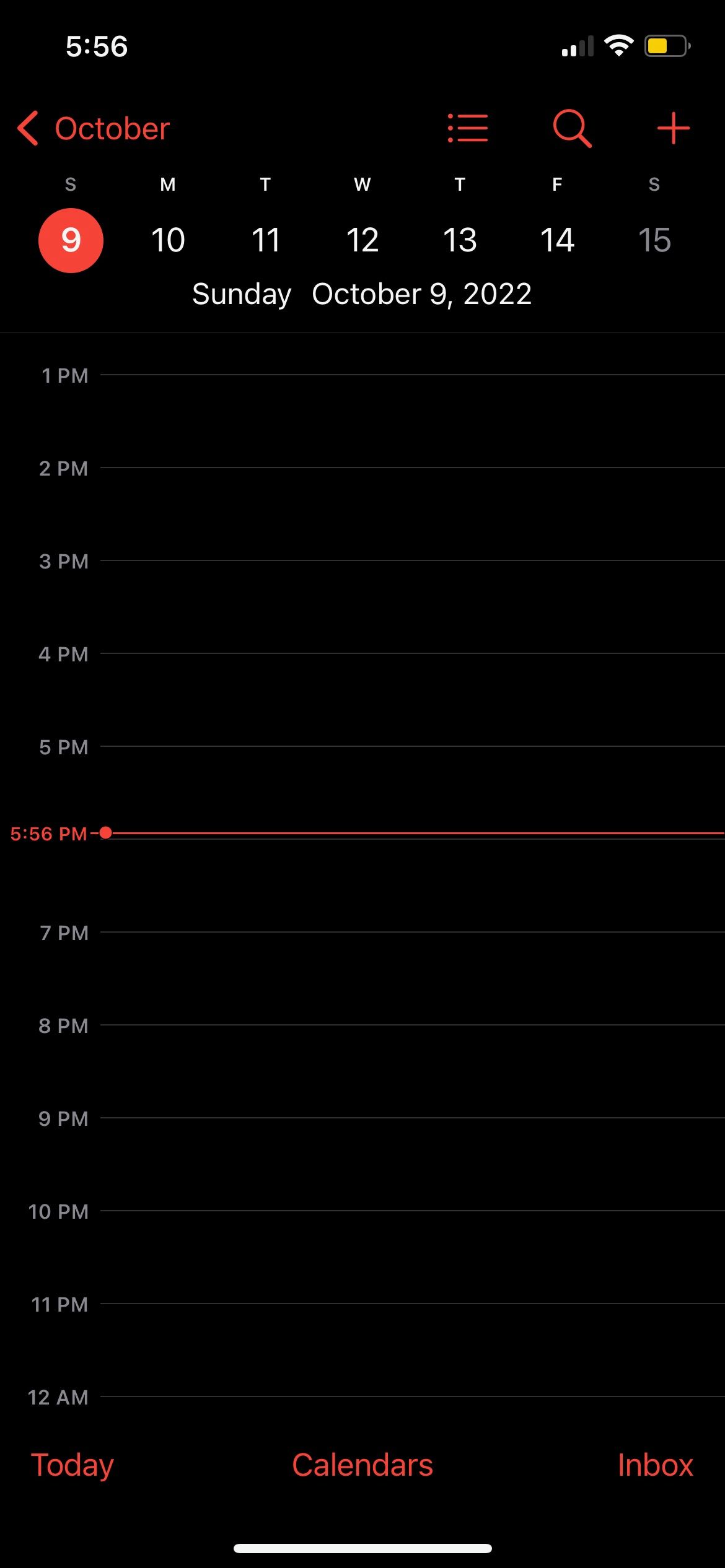This image is a screenshot taken in portrait mode with a black background. In the upper left-hand corner, the time is displayed as 5:56 PM. On the upper right-hand corner, there is an icon indicating the battery status is half-charged. Below, there is a red ‘back’ button next to the word "October." To the right, a filter icon, search icon, and a plus sign are visible. 

The calendar layout shows the initial letters of the days of the week: S, M, T, W, T, F, S. Below this row are the dates from 9 to 15. The number 9 is highlighted with a red circle. Directly underneath, it states "Sunday, October 9th, 2022," followed by hourly time slots from 1 PM to 12 AM, with 5:56 PM marked in red.

At the bottom, there are three labeled sections: "Today" on the left, "Calendars" in the center, and "Inbox" on the right. This appears to be a calendar application screenshot taken on Sunday, October 9th, 2022, at 5:56 PM, indicating no events scheduled for that day up to the current time.